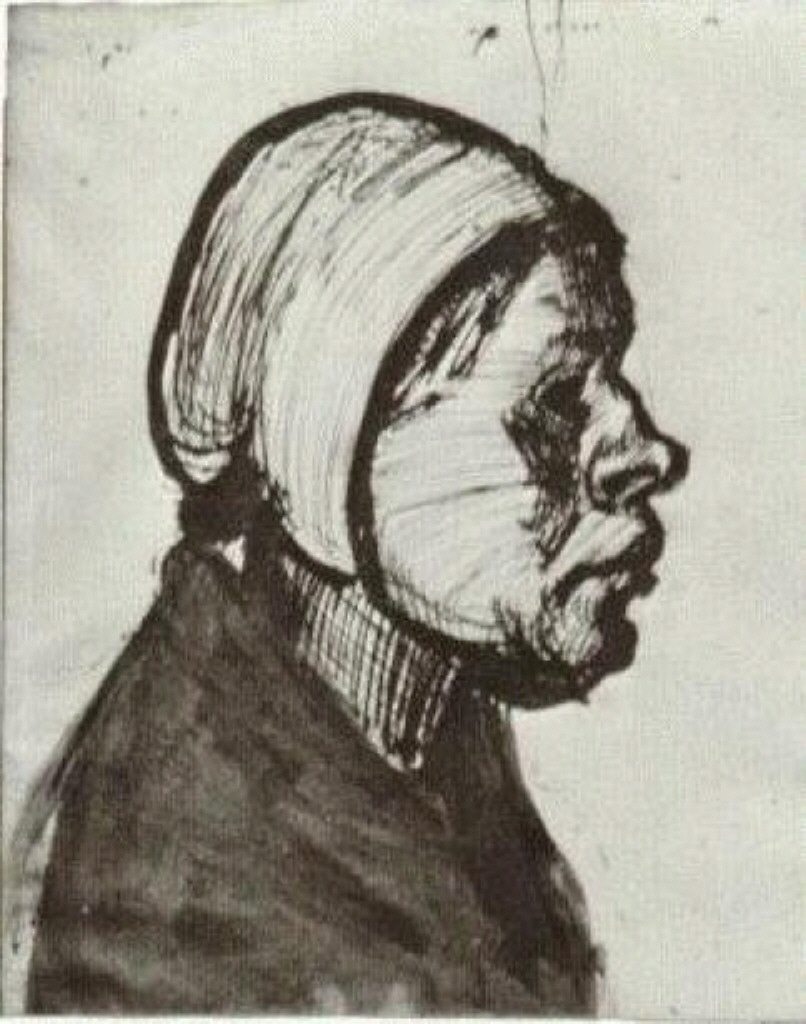The black and white sketch depicts an elderly woman from mid-torso up, facing right. Her attire consists of dark, undefined clothing—perhaps a coat or shirt—drawn with bold, black charcoal strokes, contrasting against the primarily white background with faint streaks of grey and black. Her hair is covered in a cloth tied in a babushka style scarf, with a few strands peeking out. Her face, characterized by a puffy texture suggesting age and wrinkles, shows a large, upturned nose with a crooked hump, and an almost frown-like, empty expression. The eyes are strikingly filled in entirely with black, creating a haunting, hollow look. Her neck is marked with numerous stripes, possibly indicating a high-collared neckline. Despite the basic, quick execution, the portrait captures a solemn, detailed glimpse of the woman's profile.